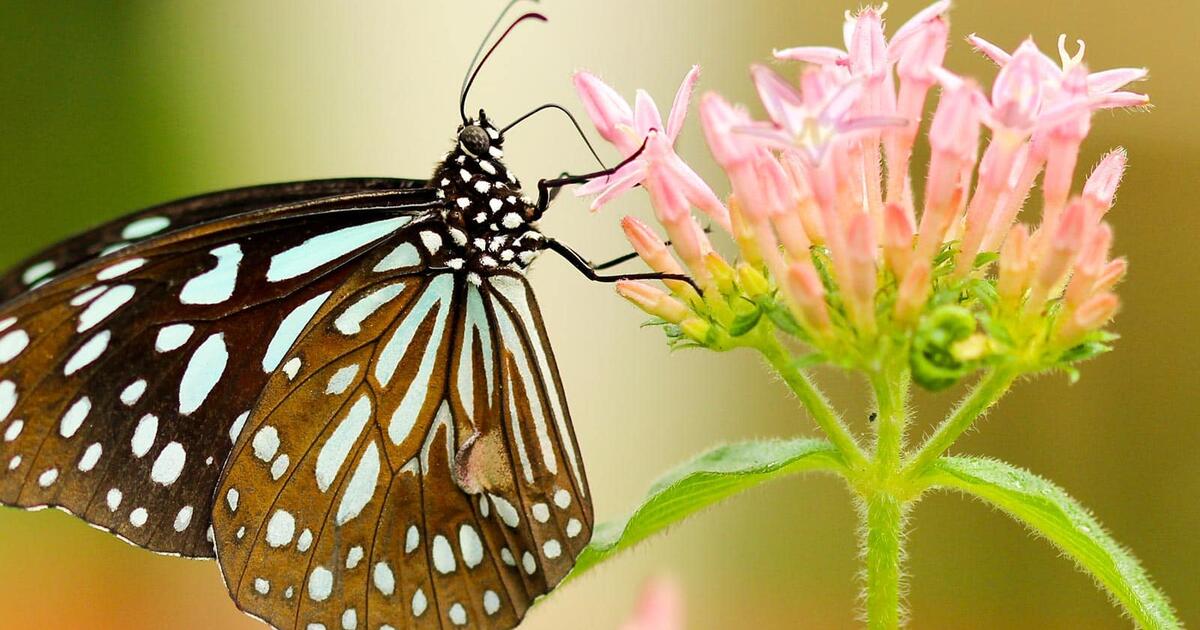This professionally taken, up-close photograph showcases a monarch butterfly in stunning detail. The butterfly features predominantly black wings adorned with very light baby blue accents, along with intricate dots and lines. Its black body is speckled with white dots and is supported by black legs as it clings delicately to a vibrant pink flower. The flower itself is bursting with light pink petals, and the green stems, covered in tiny white fuzzy hairs, further enhance the natural beauty depicted. The butterfly appears to be feeding, with its proboscis extending into the flower. The background is artistically blurred into shades of green, white, and brown, ensuring full focus on the butterfly and its floral perch. The edges of the butterfly’s wings and some leaves are partially clipped, highlighting the frame's intimate, detailed nature. Overall, the image masterfully captures the vivid colors and intricate details of both the butterfly and the flower, embodying the exquisite beauty of nature.